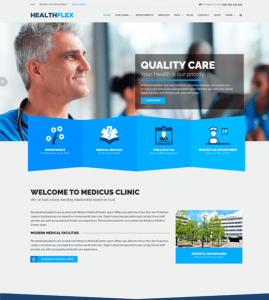**Screenshot of Clinic's Homepage Detailed Description:**

The homepage of a clinic website titled "Health Flex" is displayed. At the top, a medium grey header spans the screen. Positioned in the top left corner is the clinic's logo, with the word "Health" in dark blue and "Flex" in light blue. To the right of the logo lie the website navigation sections; the first section is highlighted in light blue while the remaining sections are grey, though the text is too blurry to read.

Beneath the header is a large background photograph featuring a man in blue scrubs. He has grey hair and is smiling warmly while looking off to the right. In the out-of-focus background are three other individuals: two women also in blue scrubs and a doctor in a white coat. They are gathered around what appears to be a clipboard.

Superimposed over this group is a translucent grey square containing large white text stating, "Quality Care. Your health is our priority." This text is underlined with a solid blue line. Below, there is more white text forming a descriptive paragraph, which is unfortunately too blurry to decipher. Under this paragraph sits a light blue button with white text.

The bottom portion of the photograph transitions into a background resembling an unfolded map, entirely shaded in blue. This section is divided into four parts, each containing a distinct white icon: a plant or tree with circles on its branches, a clinic building, a clipboard with a person's silhouette, and simply a silhouette of a person.